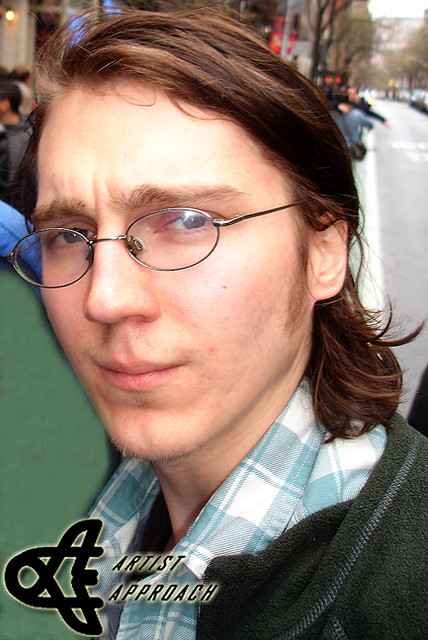The image depicts a man, standing outdoors in a bustling downtown area, positioned almost directly at the center of the frame. He is white, with long brownish hair and sideburns, wearing small oval glasses. His expression is a subtle smirk, and he is clad in a white and green checkered shirt overlaid by a gray jacket. He is resting his face against something green to the left.

The ground is an asphalt road, typical for streets where cars drive, and there are visible street markings, including a white line near the man. In the background, there are blurred trees and vehicles, along with a crowd of people gathered near some stores or businesses. The setting indicates it’s daytime. 

At the bottom left corner of the image, there is a logo with the text “Artist Approach.” The colors in the scene range from black, white, green, blue, tan, brown, yellow, pink, to red, indicating a vibrant, colorful environment. The overall orientation suggests a lively, urban atmosphere with the man as the focal point of the composition.